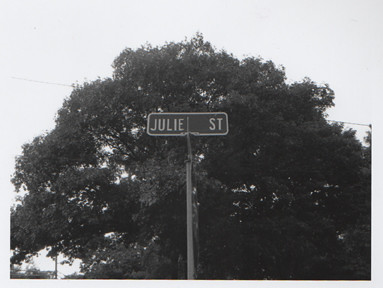The black and white photograph depicts a prominent street sign that reads "Julie Street," centered in the image. The sign, with its clear white lettering on a dark background and bordered in white, is mounted on a gray metal pole that extends off-camera. Behind the sign stands a large, bushy tree with dark leaves, occupying much of the background. A power line stretches horizontally across the upper third of the image, contrasting against a very cloudy sky. The sky appears nearly white, suggesting an overcast day. There might be the faint outline of rooftops or buildings in the lower left corner, though details are obscured by the tree. The photo is framed with a light gray border, enhancing its portrait-like composition.